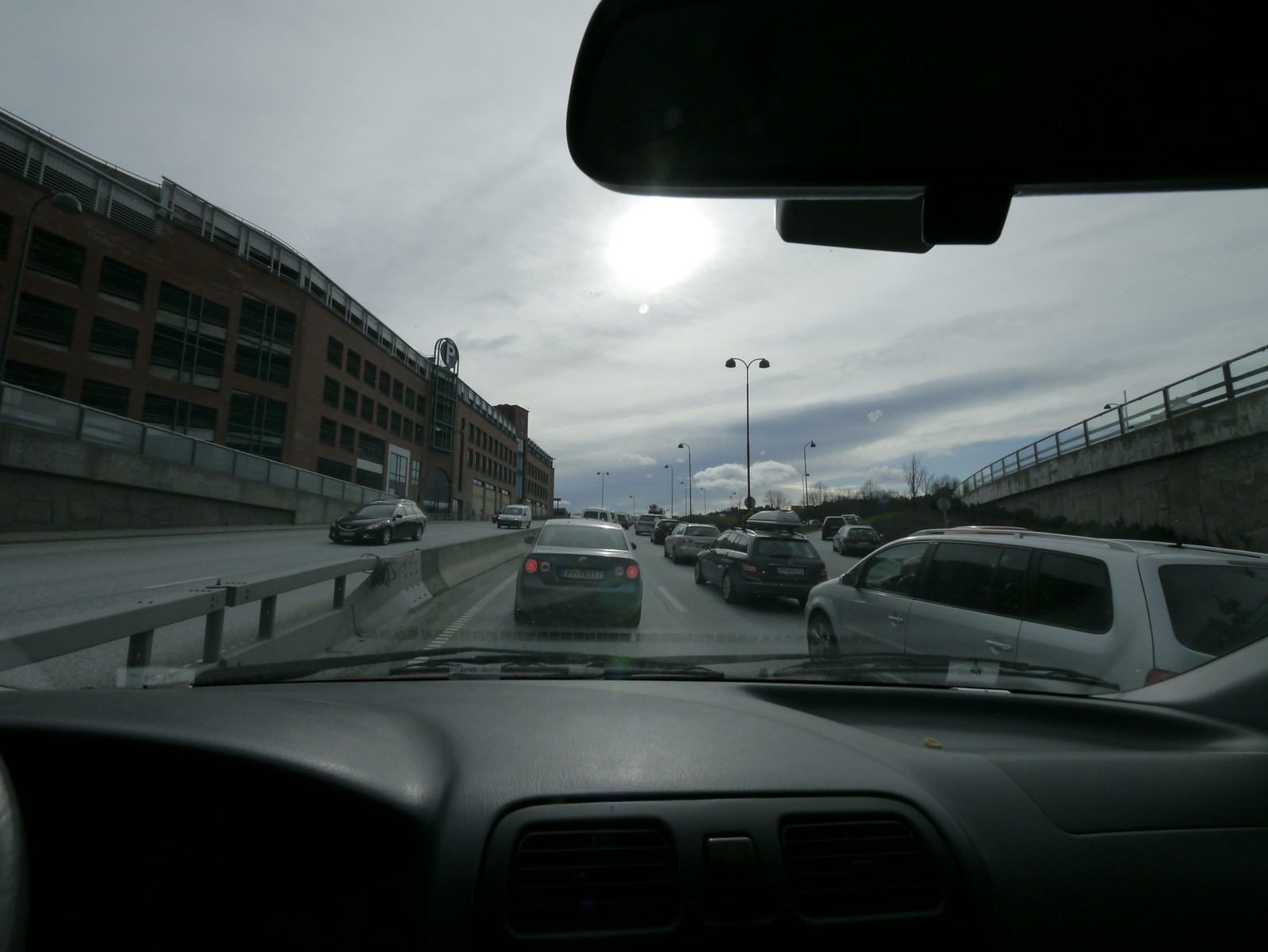The scene captures a detailed view from the interior of a relatively narrow automobile, stopped in the interior lane adjacent to a concrete and railing median. The photo is taken through the windshield, revealing an urban highway with multiple lanes. To the right, another lane is visible where vehicles, including a van immediately to the side, are merging into traffic. Ahead, a car with brake lights on suggests that the traffic is at a standstill. On the opposite side of the median, multi-lane traffic moves in the opposite direction. The sun, partially obscured by clouds, illuminates the scene with a bright yet diffused light. The car's rearview mirror, visible in the frame, reflects nothing specific from the rear. To the right, a high abutment with a guard rail implies another roadway, possibly an overpass or an elevated lane, which may be merging downwards. Approximately 100 yards ahead, vehicles appear to be exiting to the right. Buildings can be seen lining the left side of the roadway, completing this intricate urban traffic tableau.